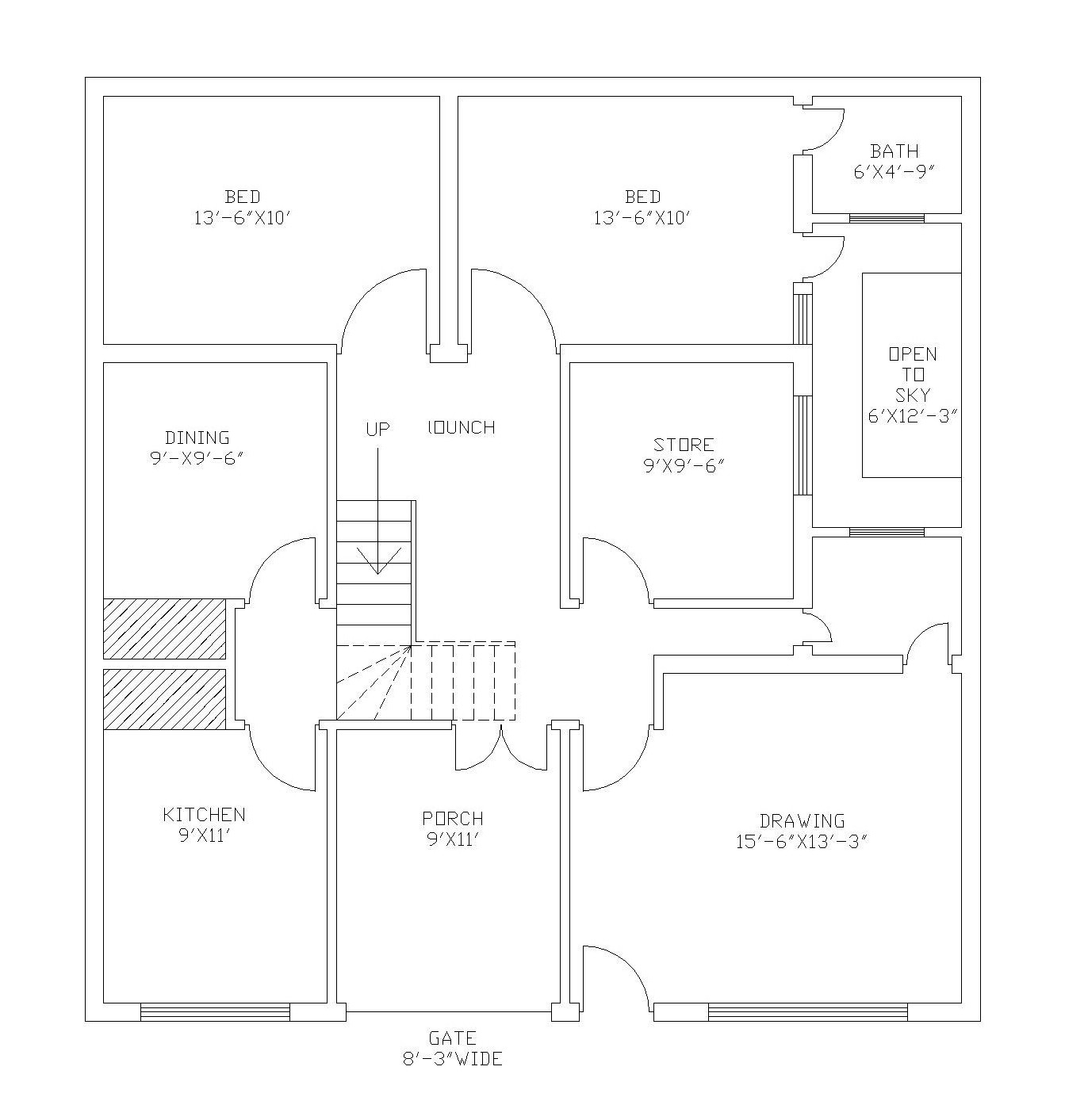A meticulously detailed black and white blueprint featuring various labeled sections. In the top left corner, it indicates "Bed 13'-6"x10'" followed by a repeated label "Bed 13'-6"x10'". The top right corner is marked "Bath 6'x4'-9"". Beneath this section, a line is drawn and labeled "Open to Sky 6'x12'-3"". Adjacent to the left, there is a section labeled "Store 9'x9'-6"". At the center of this area, an oval is enclosed with the label "I-O-U-N-C-H". Moving leftward, it states "Up" with a corresponding arrow pointing towards "Steps". Further left, a section designated "Dining 9'x9'-6"" is visible. Below this, in the bottom left corner, the blueprint marks "Kitchen 9'x11'", while to the right of the kitchen, there is a section labeled "Porch 9'x11'". To the immediate right, a large area is indicated as "Drawing 15'-6"x13'-9"". Finally, at the very bottom of the drawing, a gate is illustrated and labeled "Gate 8'x3'-Wide".